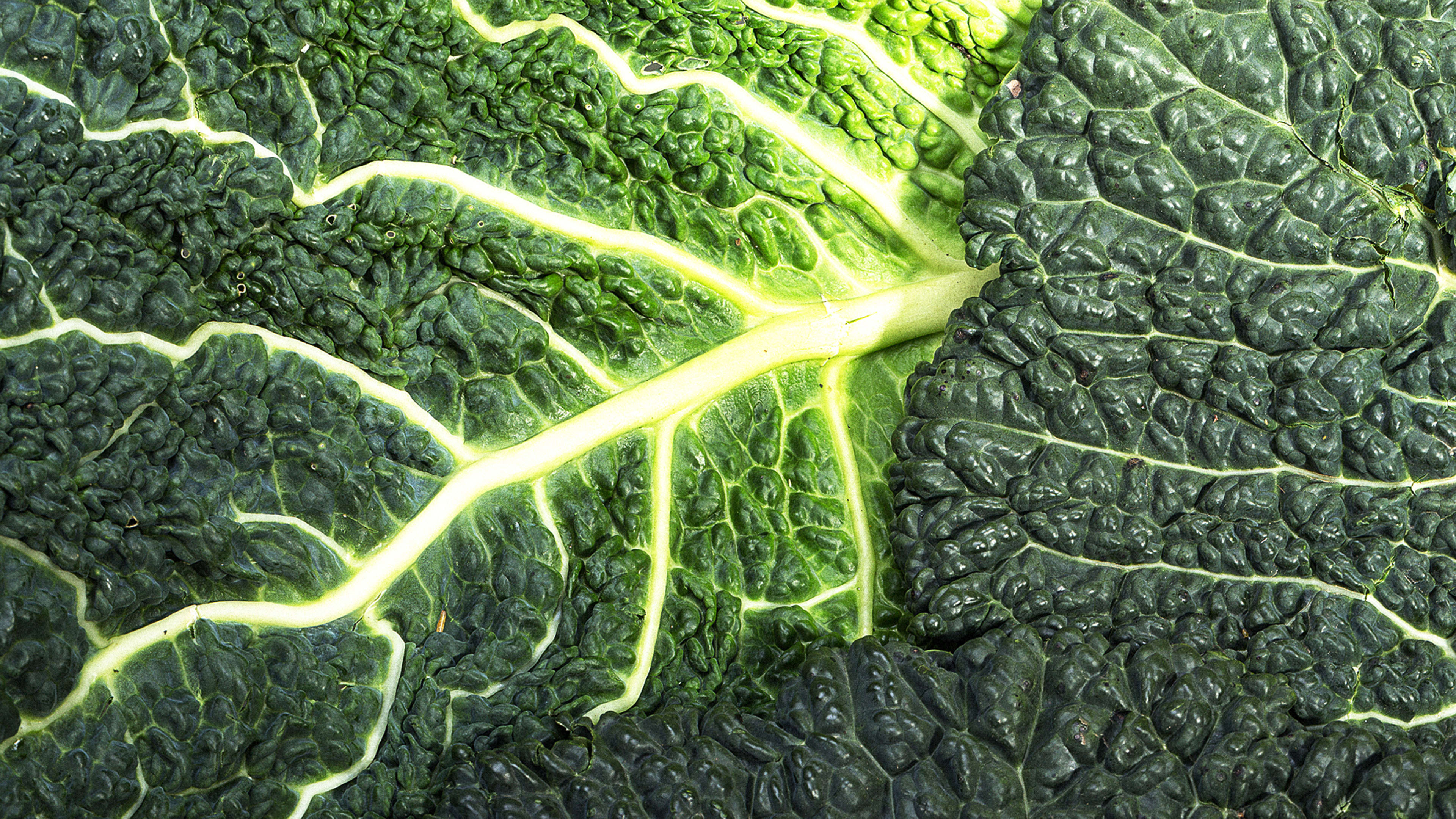This is a close-up view of a leaf, likely from kale or a similar green leafy vegetable. The image emphasizes the unique textures and colors of the leaf. The central veins are accentuated in a vibrant, almost fluorescent light yellow, transitioning to a glowing lime green near their bases. These highlighted veins create a striking contrast against the darker, textured, and bumpy green of the rest of the leaf. The right side of the leaf shows darker green tones, while the center transitions into lighter greens, and the left side exhibits medium green hues. The leaf's intricate contours, grooves, and bumps are clearly visible, giving a detailed, almost mountain range-like appearance from a top-down perspective. The leaf appears to be flat, possibly with another leaf beneath it, further emphasizing its detailed and varied texture.